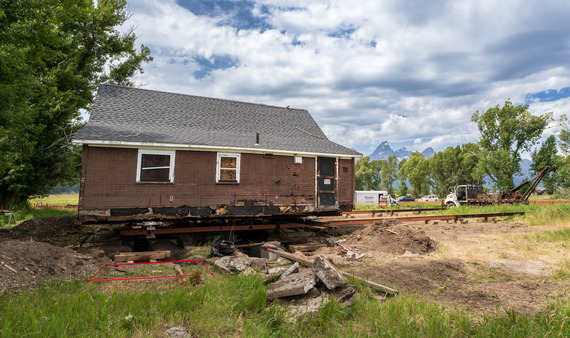This daytime photograph captures an outdoor scene featuring an old, small ranch house prominently positioned in the upper left. The house is made of brick with a newly installed gray roof and appears to have been elevated off its foundation, possibly in preparation for relocation or renovation. The house is lifted on two long metal pillars, with the ground beneath it extensively dug out, leaving dirt mounds and removed concrete blocks visible. Some of the house's brick siding has fallen off or been removed.

In the lower part of the image, green grass transitions into dirt mounds where the ground has been disturbed. A large green leaf tree stands to the left of the house.

To the right of the house, there is a collection of vehicles, including a large tow truck with white doors, a U-Haul truck, and two other rigs parked in the field. The background features additional trees and a distant mountain range beneath a mostly cloudy sky with some dark blue patches peeking through.

Overall, this scene suggests significant construction or relocation activity, highlighting the house's precarious position and the mix of natural and built environments surrounding it.